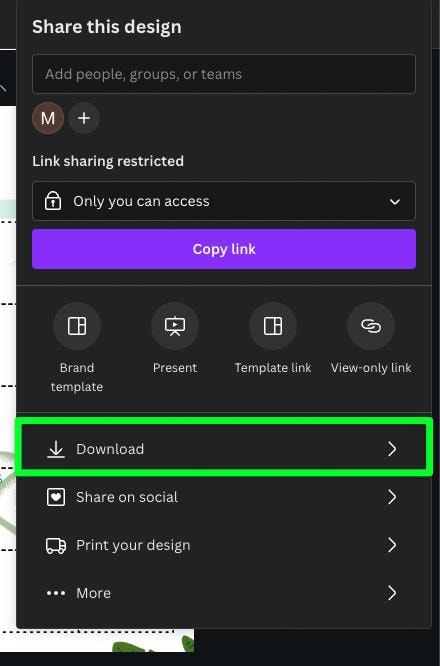This is a detailed screenshot of a design-sharing interface. The prominent element is a large vertical black rectangle situated prominently in the center. To the left and bottom edges of this rectangle, there are visible sections of a screen displaying shades of white, gray, and green.

In the upper left corner of the black rectangle, text in white reads "Share this design." Just below this text is a dark black box outlined in gray, containing the gray text "Add people, groups, or teams." 

Beneath this box, on the left side, there is a brown circle with a white capital "M" inside. To the right of this circle is a gray circle with a white plus sign. Immediately below these circles, the white text reads "Link sharing restricted."

Following this text is a black rectangular dropdown box. Inside this box, on the left side, there is a white lock icon. To the right of the lock, white text reads "Only you can access," accompanied by a downward arrow on the far right.

Beneath the dropdown box, there is a long, horizontally oriented rectangular button in a pink-purple color, with white text that reads "Copy link."

Below the pink button is a row of four icons, evenly spaced. The icons represent (from left to right): Brand Template, Present, Template Link, and View Only Link.

Further down, there is a list of three options accompanied by icons to the left of each: Download, Share on Social, and Print your design. The "Download" option is highlighted with a lime green rectangle. 

At the very bottom, there is the word "More" followed by three horizontal ellipses. Finally, on the right side of all these bottom lines, there is a right-pointing white arrow resembling a sideways "V."